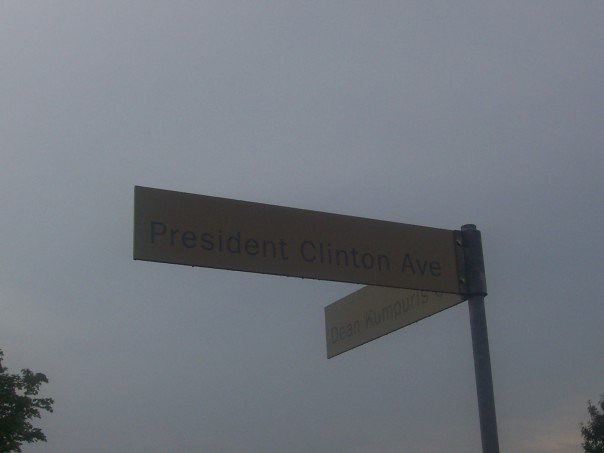A daytime photograph captures a slightly hazy, dusk-like sky transitioning from light blue to gray without any visible clouds. In the forefront, a gray metal pole supports two street signs affixed with silver bolts, forming an L shape. The sign facing left reads "President Clinton Ave," while the sign facing right appears to say "Dean Kumaris." The signs are a beige-yellow color. On the left and right lower corners of the image, green-tinged tree branches stretch into the frame, hinting at a possible residential area. Subtle hues of yellow and orange suggest the approaching sunset, adding a touch of warmth to the predominantly gray scene. The image has a slightly pixelated quality, adding to the overall haziness.